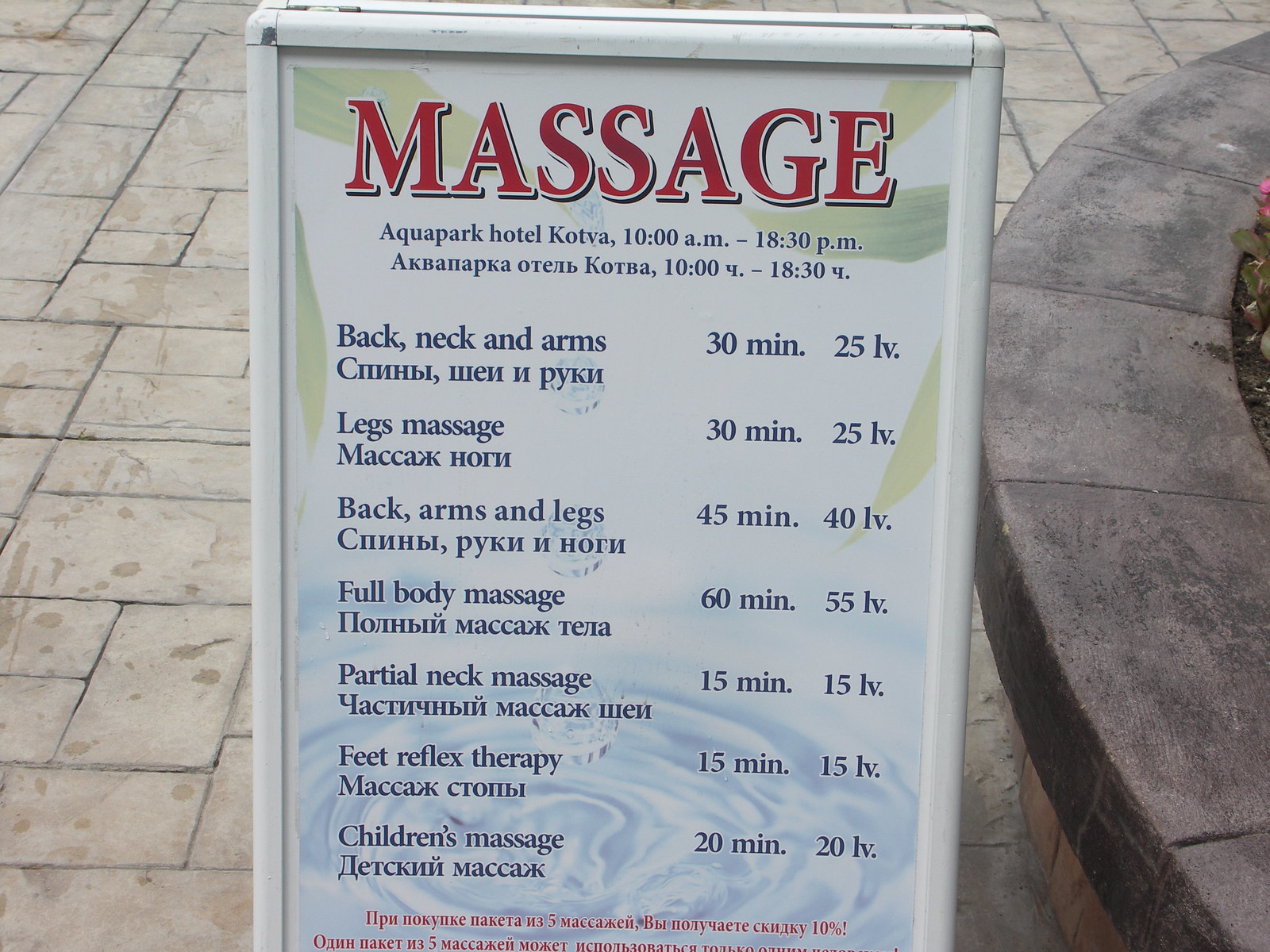The image depicts an outdoor sandwich board advertising massage services at the Aqua Park Hotel Kotva. The white, collapsible sign stands on a paved public area adorned with well-maintained city planters and a brick walkway. The sign, measuring 8 inches wide by 7 inches tall, features red text reading "Massage" at the top against a background of subtle leaves and water droplets. It offers various massage packages available from 10:00 AM to 6:30 PM, including: 

- Back, neck, and arms massage: 30 minutes for 25 LV
- Legs massage: 30 minutes for 25 LV
- Back, arms, and legs massage: 45 minutes for 40 LV
- Full body massage: 60 minutes for 55 LV
- Partial neck massage: 15 minutes for 15 LV
- Feet reflex therapy: 15 minutes for 15 LV
- Children's massage: 20 minutes for 20 LV

The text is presented in both English and Russian, making it accessible to a broader audience.